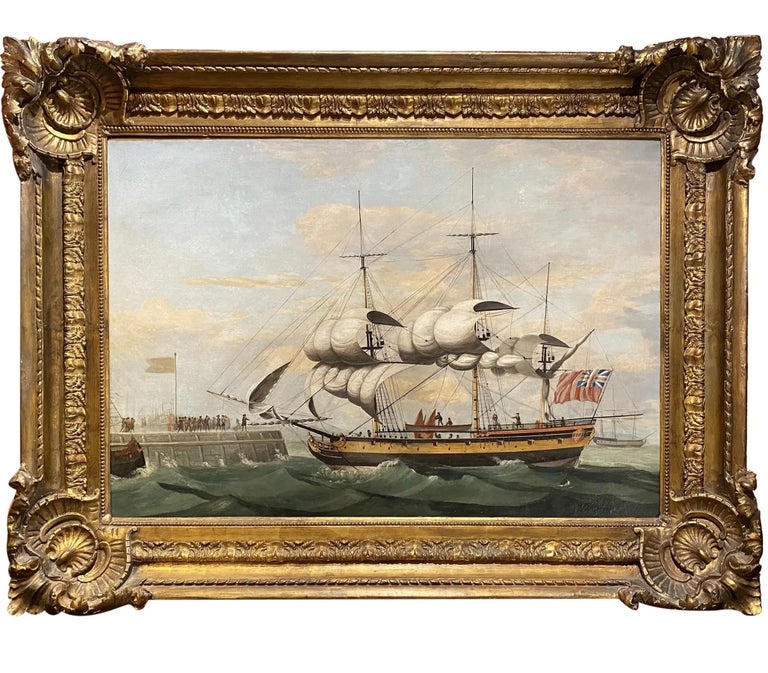The image is of an exquisitely detailed, framed piece of artwork, encased in an ornate, gold-colored frame adorned with intricate, embossed designs at each corner and along the edges. The artwork appears to be an oil painting, depicting a maritime scene. A light blue sky blanketed with wispy white and grey clouds stretches above choppy, blue-grey waves. In the foreground, a prominent ship with three billowing white sails cuts through the turbulent waters, heading to the left. The ship features a rippling Union Jack flag, indicating its British origin. Nearby, a smaller vessel with a white flag of surrender is visible, while another ship looms in the background. The scene gives an impression of an impending encounter, possibly as the larger ship approaches a distant dock populated with figures that may be soldiers.